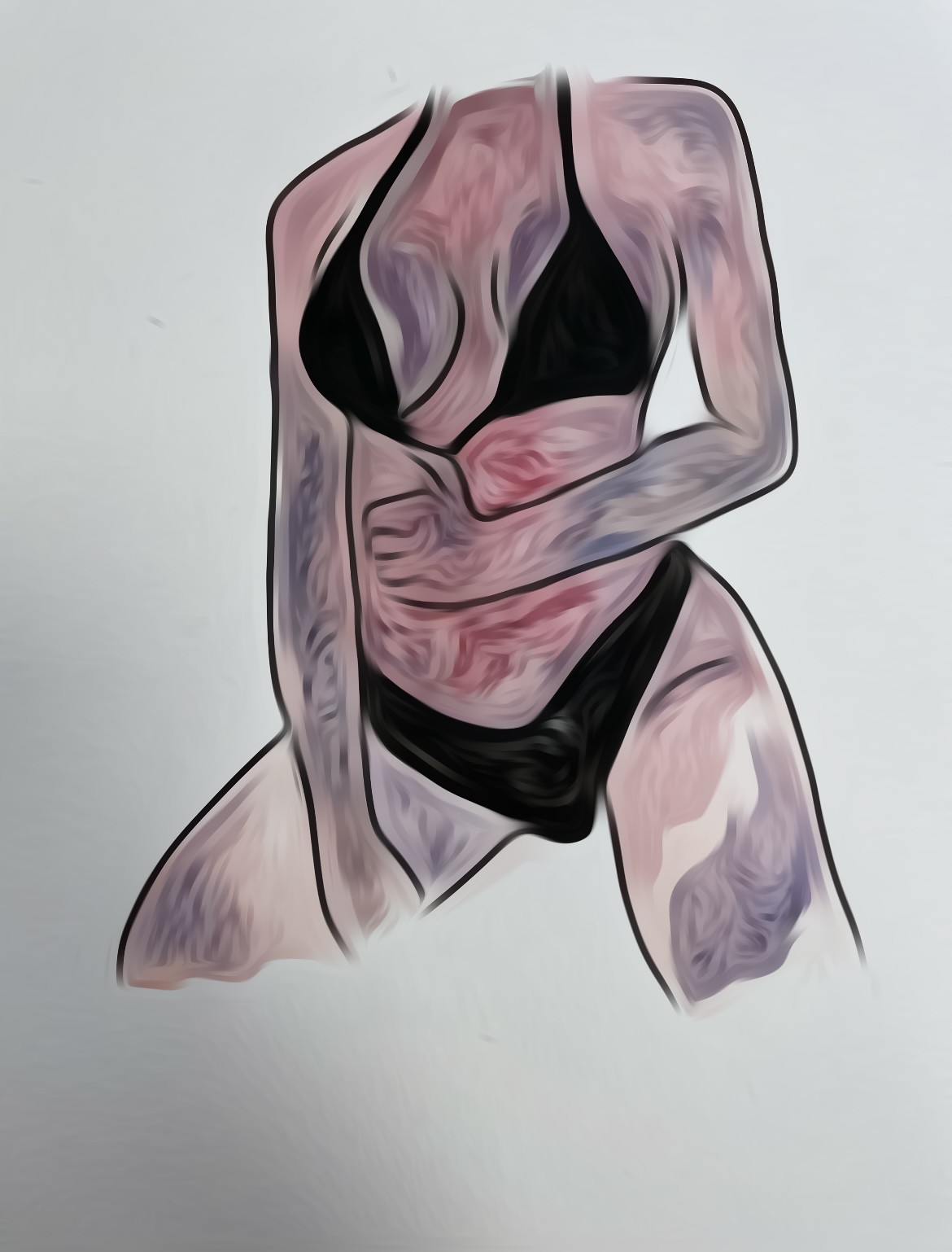This artwork depicts a woman's body, prominently centered against a stark white backdrop, creating a minimalist and striking composition. The subject is adorned in a black bikini top and matching bottoms, accentuating the various colors and forms of her body. The body's coloration is diverse: certain areas are painted in a pristine white, while others are infused with peach and reddish hues. The left hand and parts of the arms exhibit a bold black color, further contrasting the softer shades. Her thighs also feature a predominantly white tone. This juxtaposition of vivid and subtle colors across different body parts adds depth and intrigue to the artwork.